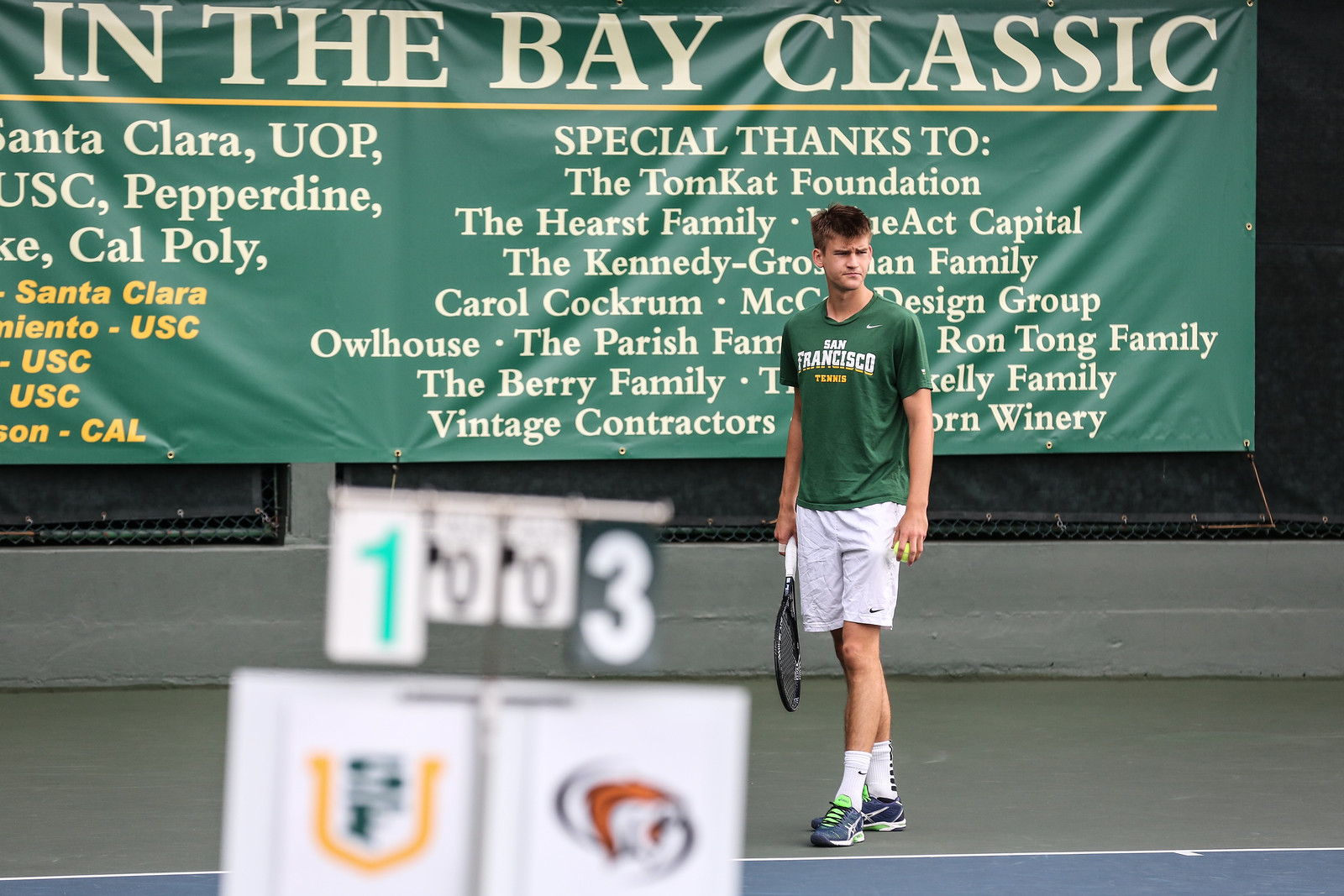The image depicts a young, white teenager, likely around 18 years old, engaged in a tennis match. He is positioned towards the center-right of the photograph, wearing a green shirt that reads "San Francisco Tennis" in white text, paired with white Nike athletic shorts, white socks, and blue shoes with green laces. The boy holds a tennis racket with a black or white handle. In the foreground, slightly blurred, stands a scoreboard showing a score of one in green and three in white. The backdrop features the back of a tennis court and a large green poster with white text that reads "In the Bay Classic." The poster lists several cities and acknowledges supporters, including: Santa Clara, UOP, Cal Poly, the Tom Katt Foundation, the Hearst family, Kennedy, Carol Cockrum, and Owl House. Their names may be partially obscured by the boy’s presence in the scene.